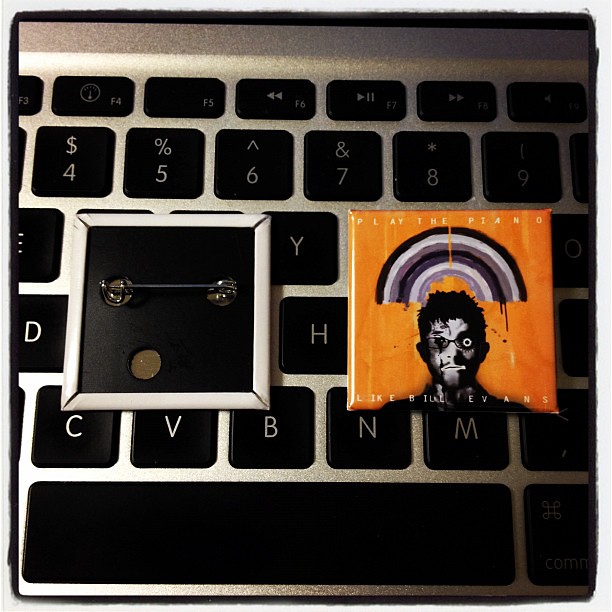This photograph, taken indoors in poor lighting, depicts a close-up of a laptop keyboard with a silver-gray body and black keys. Notably, two square pins are placed on the keyboard. The first pin, located in the center, shows its back, with a silver border and a black backing, clearly revealing the pin mechanism used for fastening to clothing. To the right, the front of a similarly sized pin is visible, featuring an enamel decoration on a burnt orange background. This decoration includes a black-and-white portrait of a man's face beneath a monochromatic black, white, and gray rainbow. Along the top of this pin, in white letters, is the phrase "Play the Piano," while the bottom text reads "Like Something Evans." The photograph's edges are outlined in black, giving it a vintage feel, and details such as function keys and the spacebar are discernable, further confirming the keyboard’s layout.